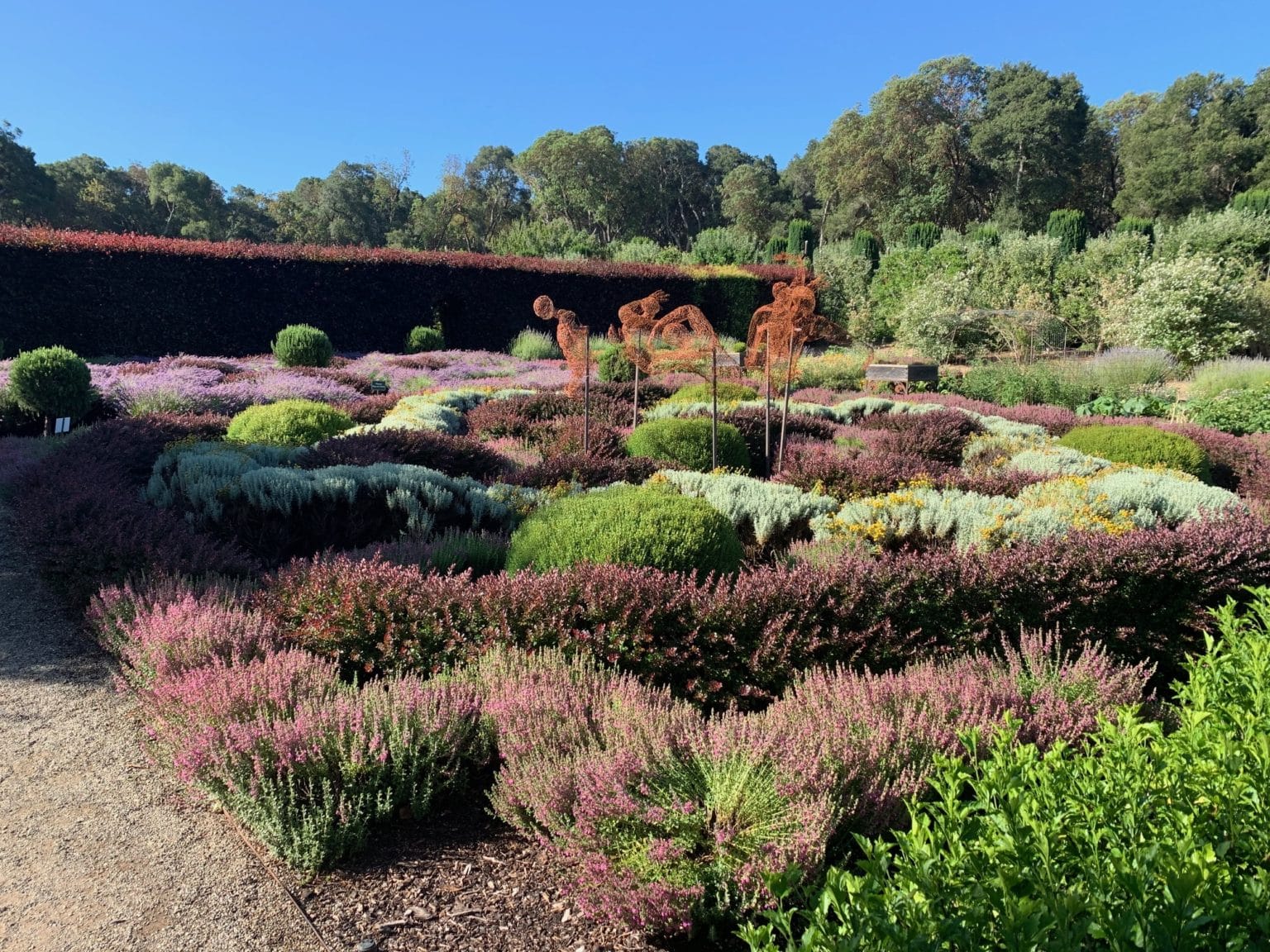This vibrant color photograph showcases a meticulously curated landscape garden bathed in sunlight under a clear, blue sky. In the background, a tree line features towering, bushy trees with lush, light green foliage, including one especially fluffy tree. An almost reddish hedge, forming a natural fence, delineates the garden's bounds, giving way to what appears to be a wooded area beyond.

The garden is artistically segmented, each area hosting distinct plant species and vibrant colors. Rounded bushes are interspersed with a mix of orange flowers, possibly orchids, along with white, pink, and purple flowers, including what seems to be lavender. Greenery includes various shades of green foliage, adding to the rich palette.

Centrally placed are intriguing metal wire structures that form part of an art exhibit. These sculptures, twisted into shapes reminiscent of human forms supported by wooden sticks, lend a creative and whimsical touch to the scene. Among the rocks and patches of dirt, the garden's carefully planned aesthetics and the array of textures and colors come together to create a serene and picturesque outdoor space.